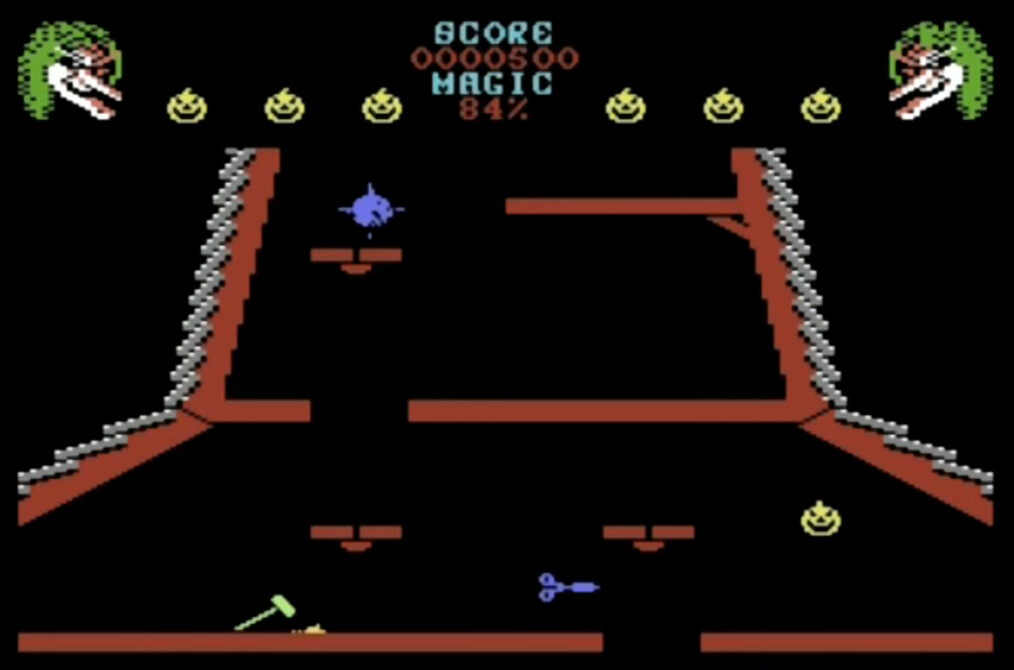This image is a screenshot from a retro horror-themed arcade game with a pitch-black background. Prominently featured in the top corners are two identical, menacing witch icons with long chins, long noses, and shoulder-length green hair, both facing inwards. Positioned between the witches, at the top center of the screen, there are three yellow jack-o'-lanterns on each side, flanking a scoreboard that displays "SCORE 0000500," followed by the words "MAGIC" and "84%". The game screen is structured with red, brick-like walls and floors, which might resemble scaffolding, and is dotted with white light bulbs along the sides. The lower right quadrant of the screen houses another yellow jack-o'-lantern, a set of purple scissors appears centrally, and a green hammer is situated near the bottom left corner. Lastly, a peculiar creature, potentially a purple shark or a blue fish, is visible in the top left corner.